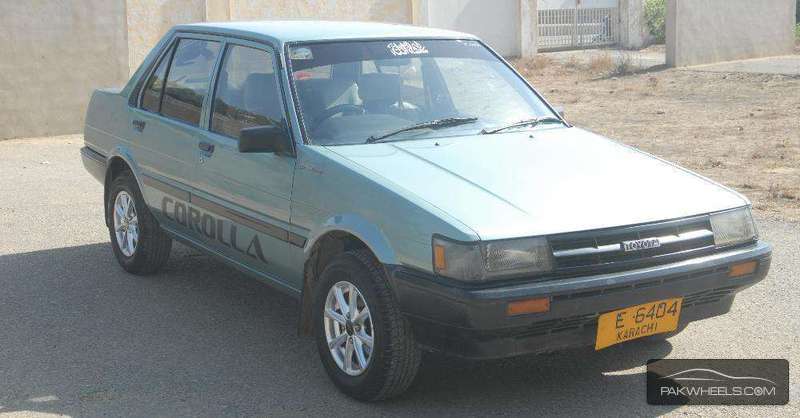The image portrays a light blue Toyota Corolla in a parking lot, angled slightly to the left while facing forward. This compact four-door vehicle, which appears to be in good working condition with no visible dents, rests on four black wheels. The front features a black bumper and is adorned with a yellow license plate that reads "Karachi E.6404." The Corolla emblem is located beneath the two front doors. Noteworthy details include black headlights with white and orange lights, and a black rectangular item on top of the windshield. The background features a tan wall with a gate, and the car is parked on cement next to a patch of dirt with dead grass. At the bottom right corner of the image, the text "PaxWheels.com" accompanied by a car silhouette is visible, suggesting this may be a listing from the website.